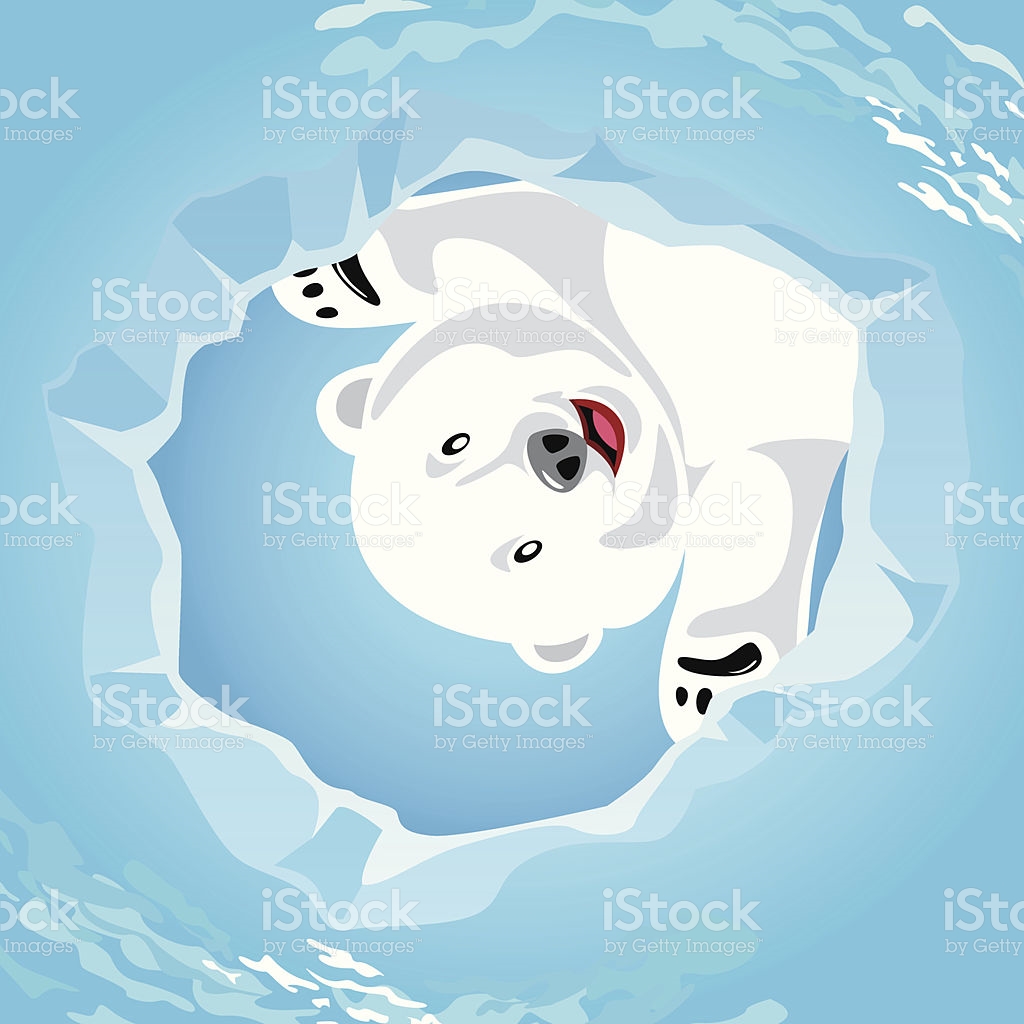In this vibrant and whimsical image, a cartoon polar bear is depicted as peeking happily down through a jagged hole in the ice. The bear's fur is predominantly white but exhibits gray shadows on its face, arms, and ears, giving it a textured appearance. Its nose is gray with black nostrils, and it has black eyes. The bear's mouth is open in an endearing, smiling expression. The bear appears to be upside down and sideways, adding a playful element to the scene. The backdrop consists of light blue snow with darker blue shades indicating depth and the gap in the ice. Only the bear's head and short paws are visible, suggesting it is curiously gazing into the hole, perhaps at its reflection. Overlaid on the image, there is a faded watermark that reads "iStock by Getty Images," contributing to its digital copyright protection. The overall composition evokes a sense of Arctic adventure and warmth through the bear's joyful demeanor.